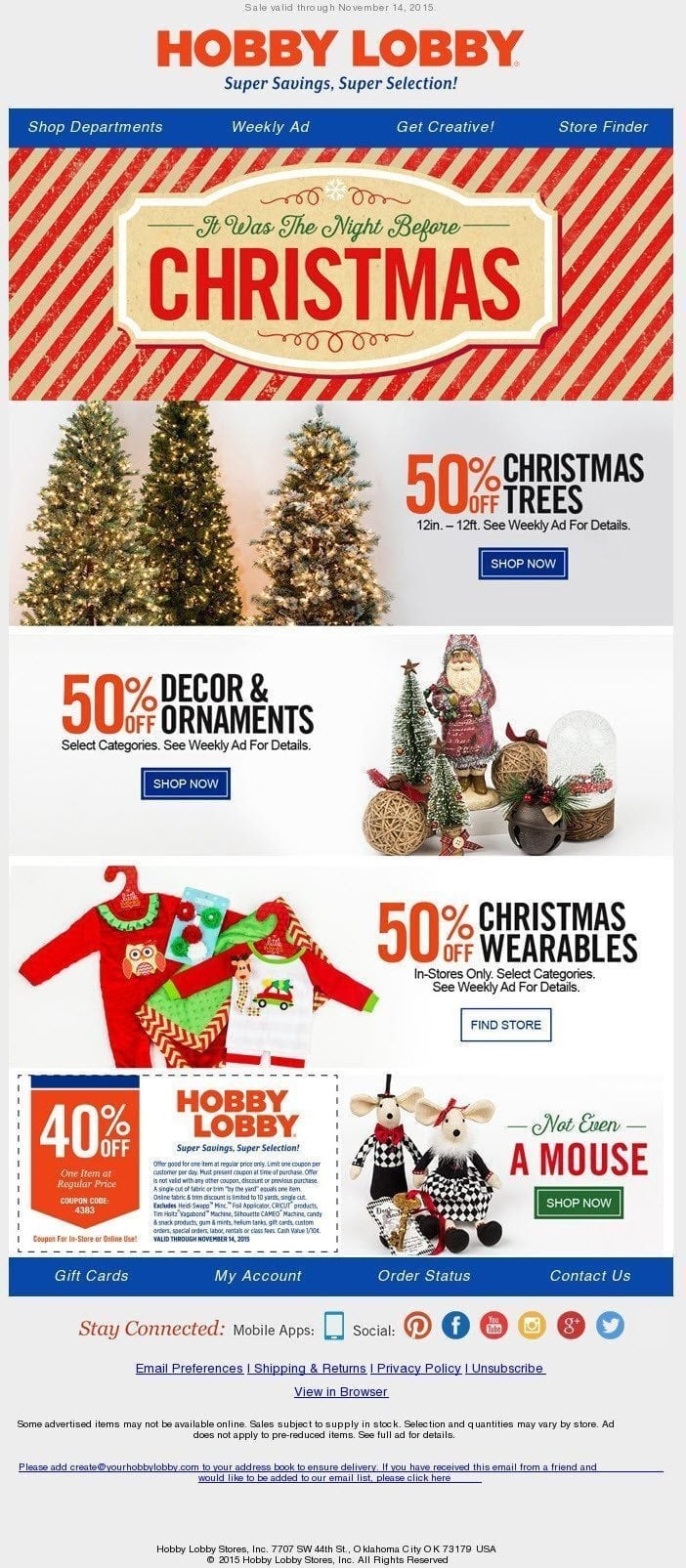This image, taken from Hobby Lobby, showcases a vibrant advertisement banner for the craft store. At the top, the "Hobby Lobby" logo is prominently displayed in bold red letters against a clean background. The banner announces a sale valid through November 14th, 2015. 

Beneath the logo, the phrases "Super Savings, Super Selection" are prominently featured, capturing the essence of the deals available. A blue rectangle runs horizontally across the middle of the banner, containing navigational prompts: "Shop Departments," "Weekly Ad," "Get Creative," and "Store Finder."

The background of the banner includes a striped red and beige design running diagonally. Superimposed on this backdrop is a beige sign with the phrase "Twas the night before" written in festive green cursive, followed by "Christmas" in bold red letters.

Towards the lower half of the banner, there's a section dedicated to Christmas sales. On the left, an image depicts three beautifully lit Christmas trees. Adjacent to this, text in bold red announces: "50% off Christmas Trees, 12 inch to 12 foot. See weekly ad for details," accompanied by a "Shop Now" button. Below this, additional offers are displayed: "50% off décor and ornaments. See select categories. See weekly ad for details," followed by another "Shop Now" button.

Further down, the banner showcases several festive figurines, including Santa Claus, Christmas trees, and a snow globe. It finishes with another promotion, detailing a 40% off Hobby Lobby coupon, inviting shoppers to take advantage of the savings.